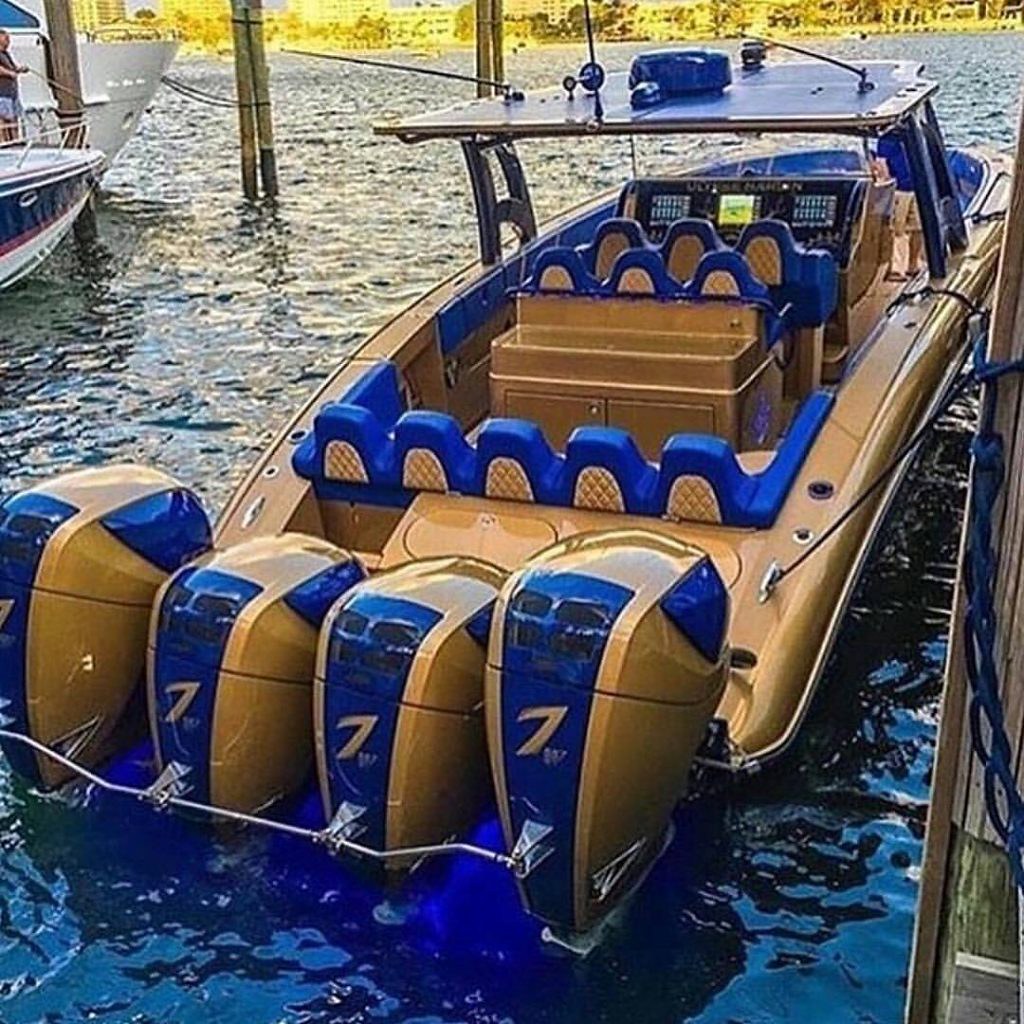This is a square color photograph of a gold-colored speedboat, docked by the water. The boat, measuring approximately 20 to 25 feet in length, features a luxurious design with seats for up to eight people. Its prominent center console is sheltered by a flat-paneled roof. The seating arrangement includes five high-backed cushioned seats in the rear, upholstered in blue, with additional seating towards the front.

The boat is equipped with four massive outboard motors at the stern, all painted in the same distinctive gold hue with blue trims and emblazoned with the number seven. The motors' striking appearance complements the boat's overall tacky but eye-catching aesthetic.

In the background, we can see a tourist resort, with hotels and apartment buildings by the sea. The setting appears to be a waterway, likely part of an ocean, lake, or river, with a couple of other boats tied up nearby. The rich details and vibrant colors make this photograph a vivid portrayal of leisure and nautical luxury.